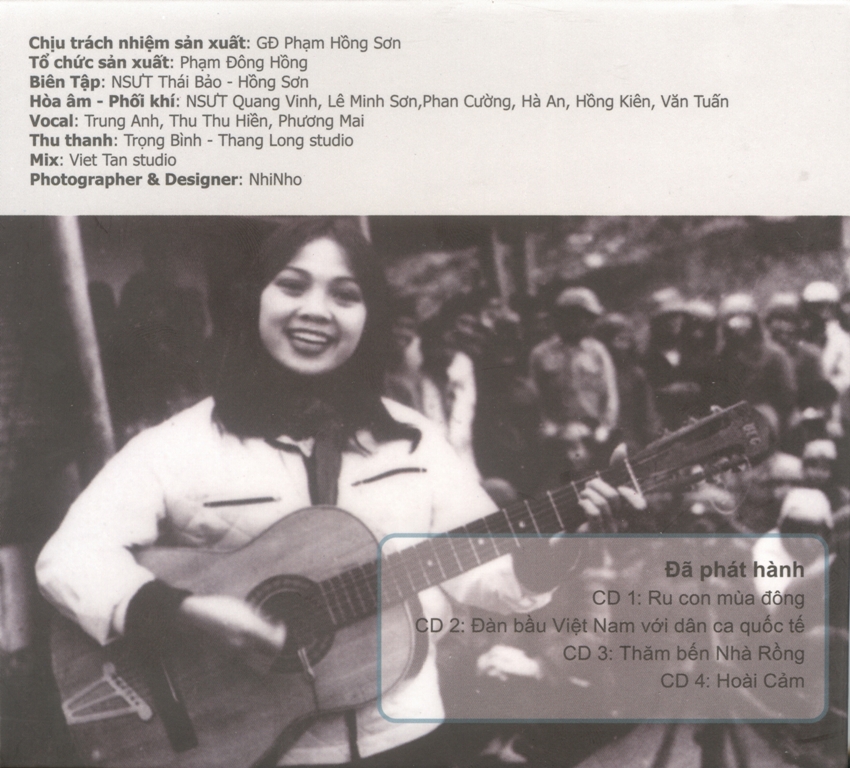In this vintage black-and-white photograph, a smiling woman with shoulder-length dark hair stands prominently, playing a guitar. She is dressed in a white jacket with pockets on the front. Her right hand is captured in motion as she strums the guitar, while her left hand holds the chords. The scene appears to be set on a stage or in front of a backdrop depicting a crowd of people, many wearing hats, possibly indicating a historical or cultural gathering. The photograph is framed by text in a foreign language that is not easily legible, with some legible phrases such as "mix studio" and "photographer and designer." The overall composition suggests a possible setting in the Philippines, adding a layer of cultural context to the image.